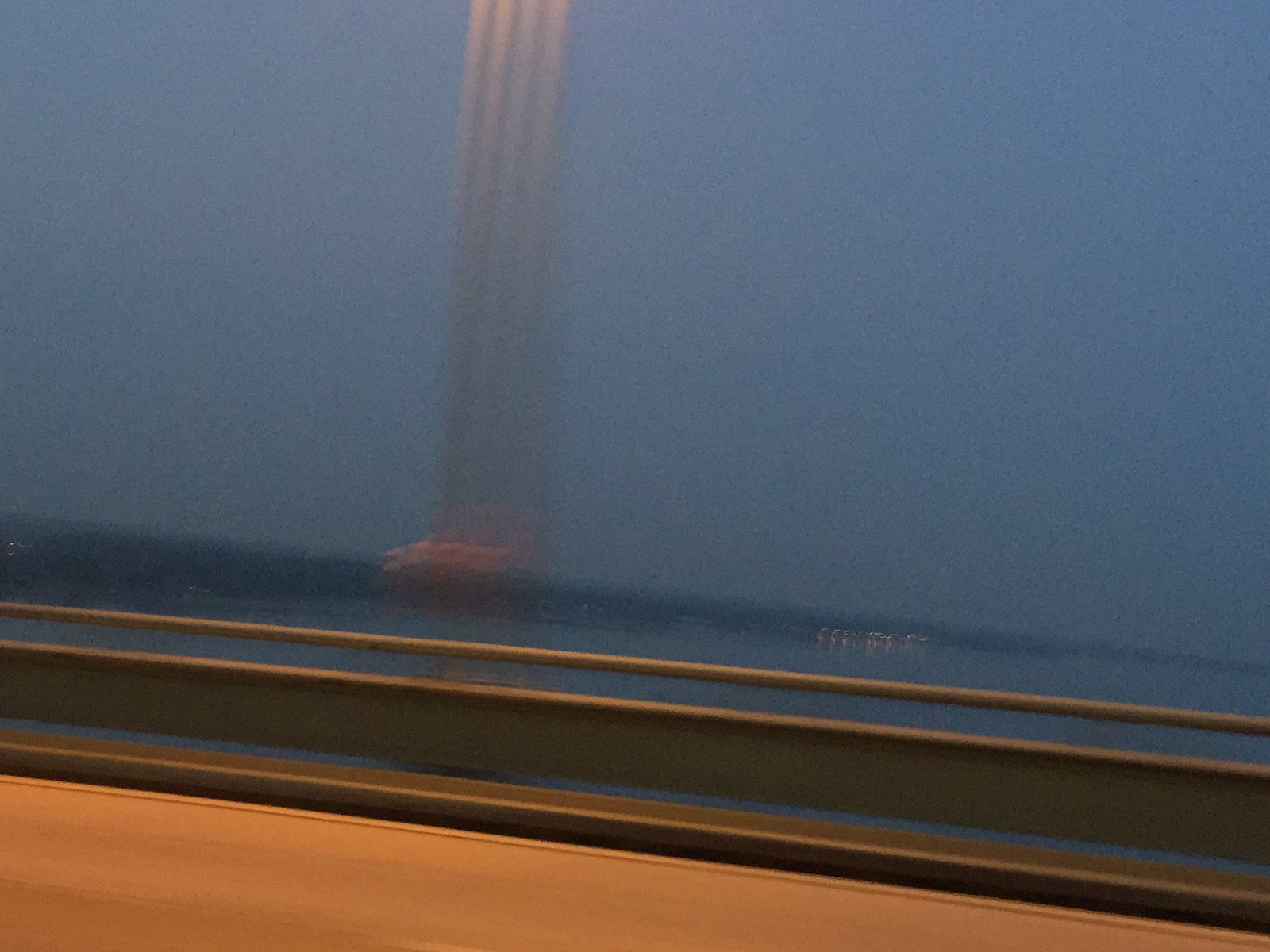Through a silver-railed window, the captivating view reveals a vast expanse of deep blue water, possibly an ocean or a river, stretching out to the horizon. The scene gives the impression of being aboard a train or rail car, journeying across the waterway. Subtle markings on the window add a touch of texture, potentially reflecting a nearby tall structure. It appears to be dusk, as the sky is gently transitioning towards darkness, providing just enough light to illuminate the shimmering water. In the distance, a few scattered lights twinkle, adding a hint of life to the tranquil scene. The image evokes a sense of peaceful movement toward an unknown destination.